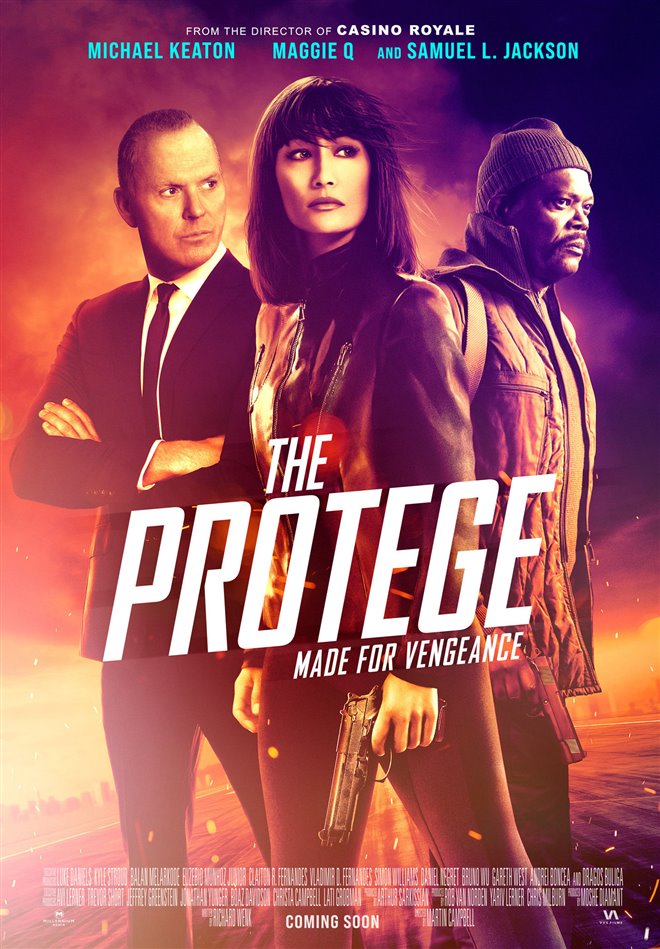This is a vibrant movie poster for the film *The Protégé*, prominently featuring the tagline "Made for Vengeance." The design employs a striking combination of purples, yellows, reds, and pinks, with white lettering for the main text and blue for the cast names. At the top, it states "From the Director of Casino Royale."

The poster showcases three main characters: Michael Keaton, Maggie Q, and Samuel L. Jackson, their names displayed in teal blue text. Michael Keaton, on the left, wears a black suit with a white shirt and black tie, exuding a serious demeanor. Positioned in the center, Maggie Q sports a sharp long bob haircut and an action-ready look, holding a black pistol and clad in a leather jacket and black pants. To the right stands Samuel L. Jackson, appearing rugged in a black stocking cap, black jacket, and a backpack, also armed with a pistol. 

All three characters face to the right, adding a sense of dynamism to the composition. Below the title, "The Protégé," is the tagline "Made for Vengeance" in smaller white letters, and at the bottom of the poster, it says "Coming Soon." The intricate interplay of bold colors and serious expressions sets the tone for this action-packed film.